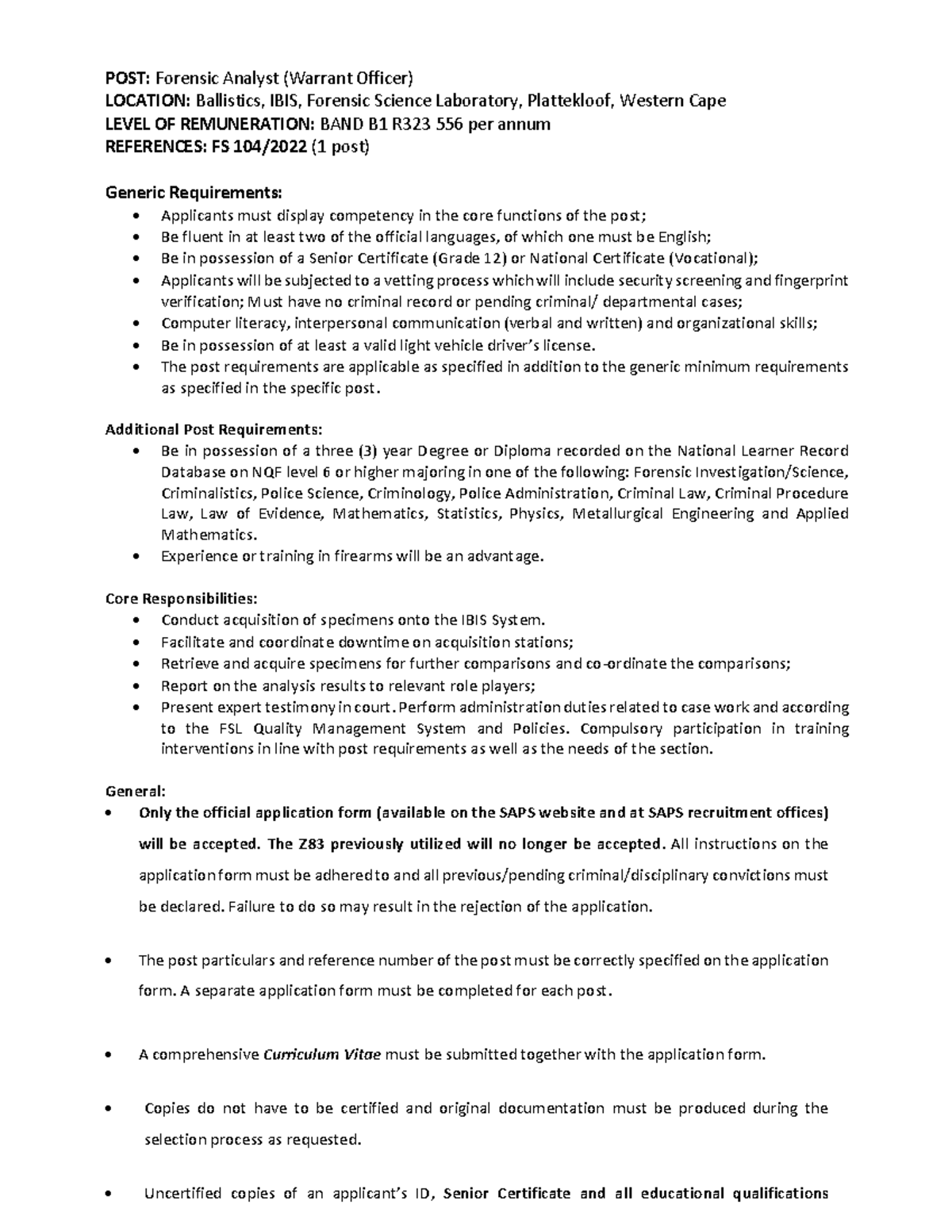The image features a job posting set against a white background with prominent black text positioned in the upper left corner detailing key information in bold. The heading reads "Post: Forensic Analyst (Warrant Officer)" followed by the next line specifying the "Location: Ballistic IBS, Forensic Science Laboratory, Plattecliffe, Western Cape," and further down, "Level of Remuneration" and "References" are mentioned.

Underneath, the caption "Generic Requirements" is highlighted in bold black text, with bullet points listing the necessary qualifications: 
- Applicants must display competency in the core functions of the post.
- Be fluent in at least two of the official languages, one of which must be English.
- Be in possession of a Senior Certificate (Grade 12) or a National Certificate (Vocational).

Continuing further, additional post-specific requirements are provided, also in bullet-point format:
- Be in possession of a three-year degree or diploma recorded on the National Learner Record Database at NQF Level 6 or higher, majoring in one of the following fields: Forensic Investigation Science, Criminalistics, Police Science, Criminology, Police Administration, or Criminal Law.

The layout is clean and neatly organized, emphasizing the necessary qualifications and educational background for potential applicants.